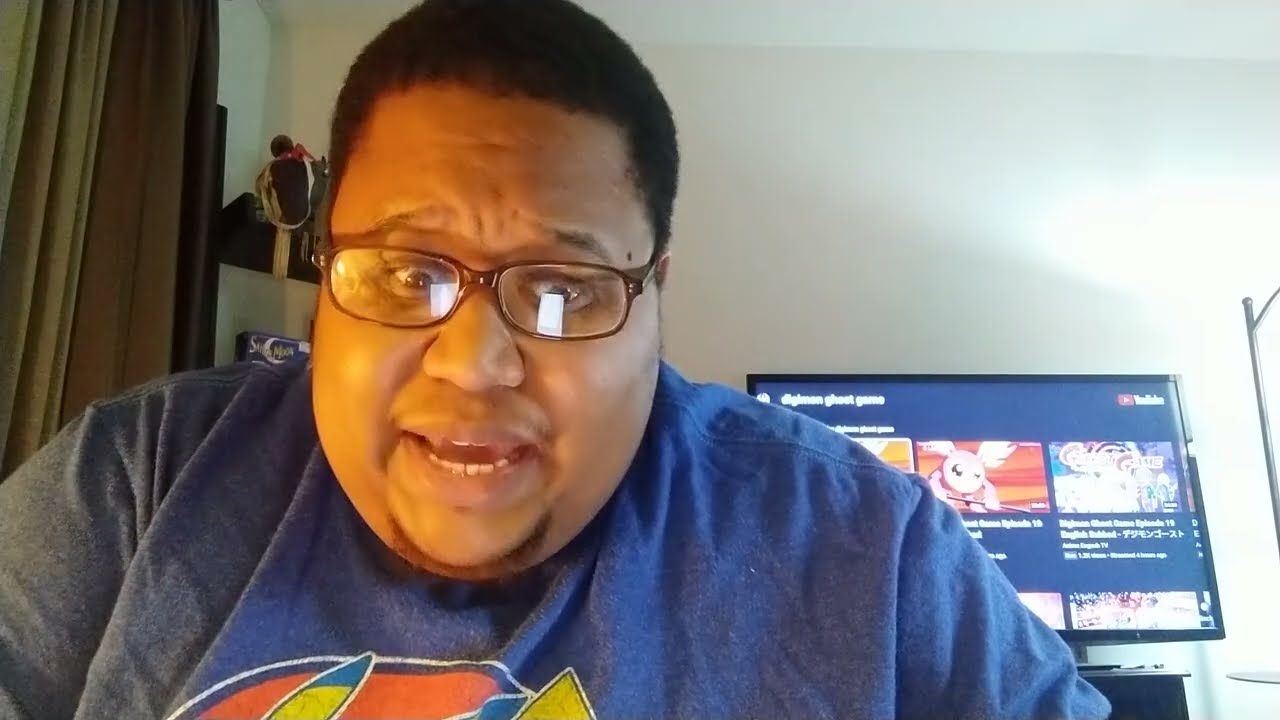The photograph is a detailed color interior shot of a man who appears to be surprised or concerned, occupying most of the screen directly in the center. He is looking down at something, which from the reflection on his dark-rimmed glasses, appears to be his phone. The man has short, curly, dark hair, a chin-only beard, and is wearing a blue cotton t-shirt featuring Pikachu from Pokémon, identifiable by the yellow and black ears and tail on the shirt. His skin appears fairly dark, suggesting he may be African-American, and he has a slightly heavy-set build.

In the background, the setting appears to be his apartment. There's a beige wall with shelves holding various items, including a Sailor Moon figurine, and a dark green curtain on the left. Behind him is a TV displaying a YouTube screen with the search bar reading "DLGLMAN Ghost Game," showing previews of animated videos. On the right, a bright white lamp illuminates the scene.